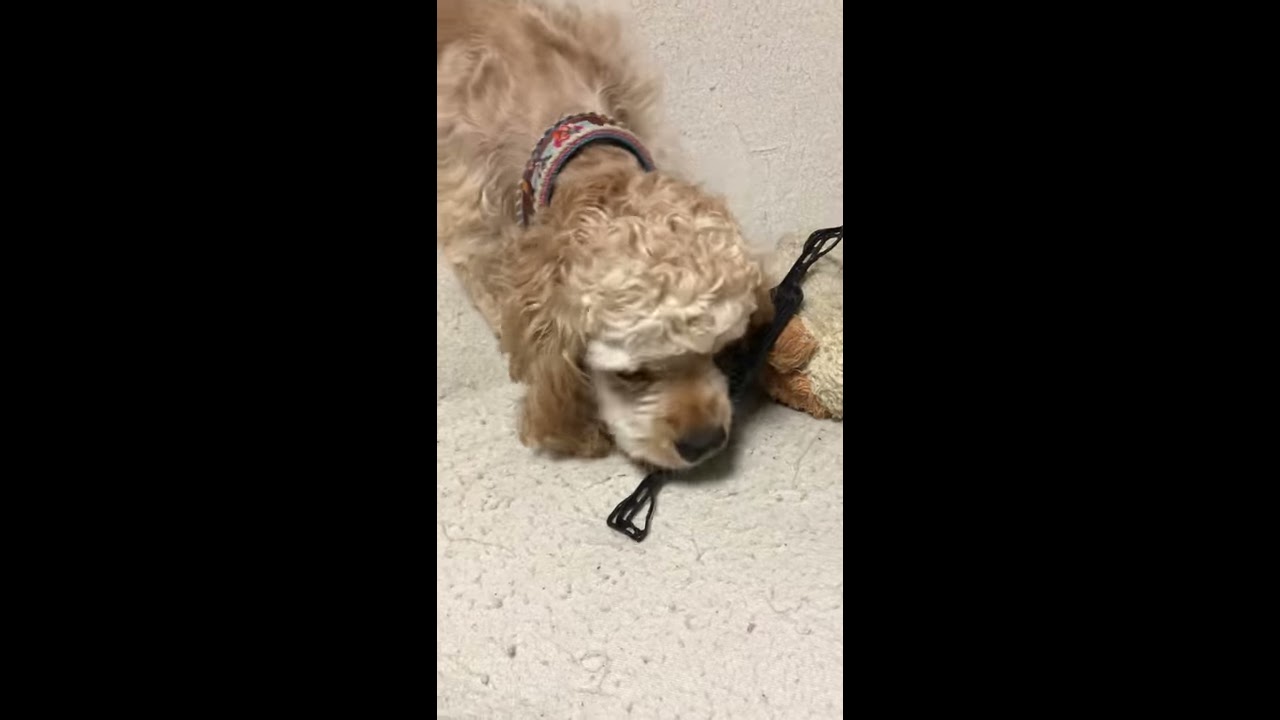The image features a medium-sized puppy, likely a Poodle, with light tan or golden, fluffy, and curly fur. The puppy lies comfortably on a white or off-white carpet, appearing thoroughly exhausted, possibly after a walk. His head rests on his front paws, one of which is draped over a black, fabric toy resembling rectangular strings. His eyes are nearly closed, suggesting he could fall asleep at any moment. The pup sports a loosely fitted, multicolored collar decorated with red flowers. There's also a leash attached to his collar, partially tucked under him. The background includes black rectangles on either side, framing the serene scene.